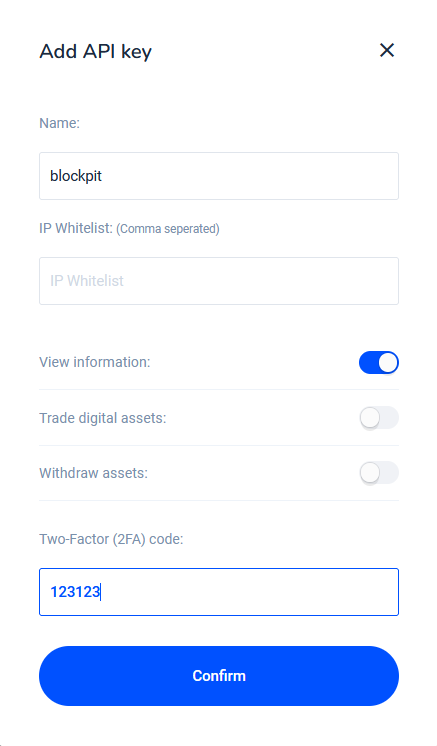The image displays a particular section of a website for adding an API key, likely viewed on a narrow screen, possibly a smartphone. At the top of the image, there is a title in black text reading "Add API Key" accompanied by a black 'X' icon, indicating an option to close the window or modal.

Below the title, there is a label "Name" with a corresponding value "Block Pit." Underneath, there is an input field labeled "IP Whitelist, comma-separated," suggesting that users can input multiple IP addresses, separated by commas. 

Further down, there is a toggled switch button in blue marked "View Information," which is turned on. Two other toggled switches labeled "Trade Digital Assets" and "Withdraw Assets" are both in the off position.

Below these settings, there is a section labeled "Two-Factor Authentication (2FA) Code," with a blue box containing the placeholder text "123123." This is followed by a long, horizontally-oriented button with rounded edges, filled with blue color and white lettering that reads "Confirm."

The entire interface is set against a plain white background, giving it a clean and minimalistic look, devoid of any grid lines or additional decorations. The layout is compact, suggesting that the image might be a screenshot of a mobile version of the website.